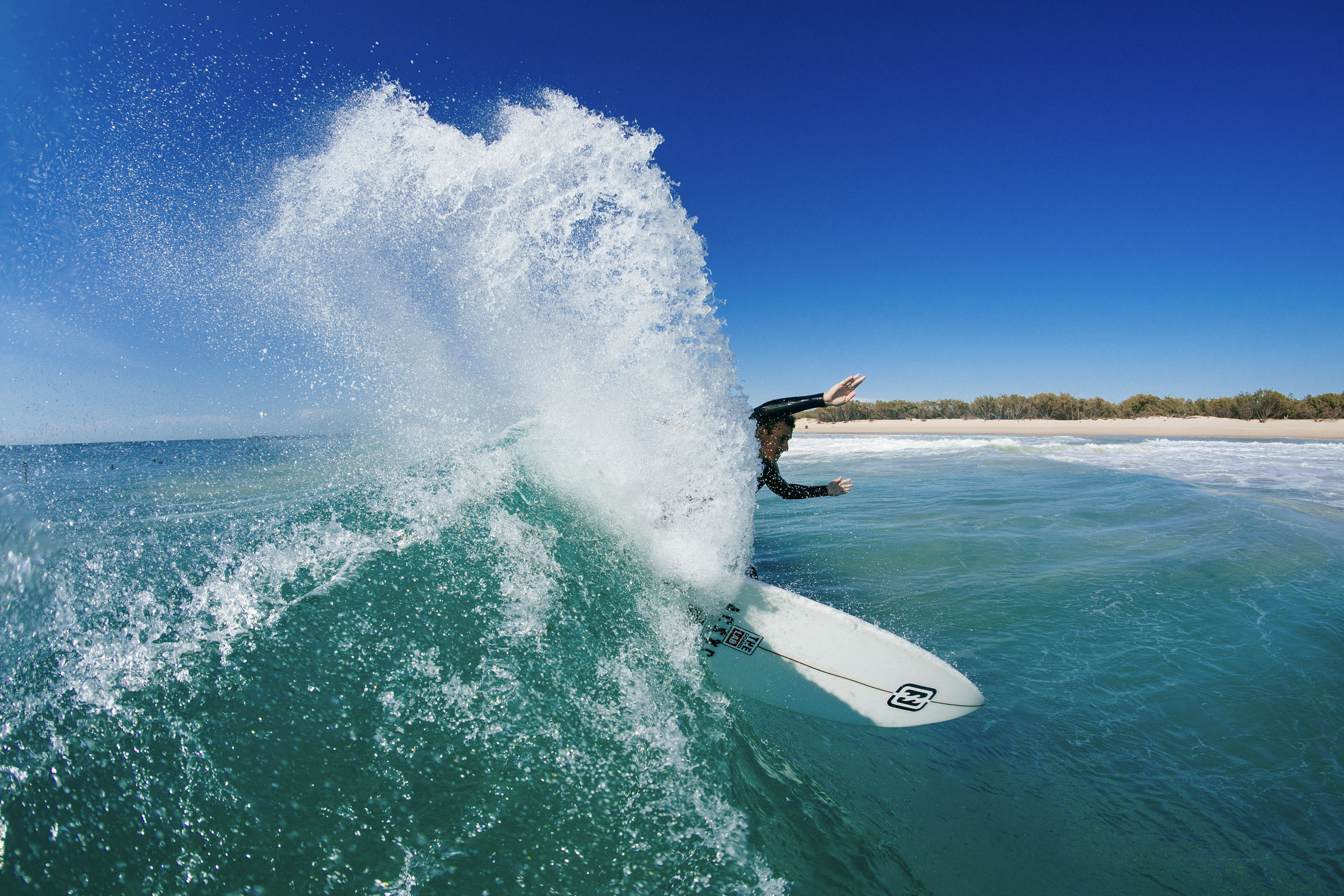The image is a realistic, horizontally oriented photograph taken during a clear day with a bright blue sky. Dominating the scene is an oceanic action shot where a man, likely in his 20s or 30s and wearing a black wetsuit, is surfing on a white surfboard adorned with unreadable black text. The surfer is in a precarious position, partially obscured by a crashing wave, with only his head and arms visible above the frothy seafoam. The cresting wave, a dynamic mix of greenish-blue water and white foam, propels him forward, creating an impression that he might be either skillfully maneuvering a turn or about to wipe out. The background features a small island or coastline to the right, with sandy shores and patches of green trees, adding depth to the overall composition. The clear, cloudless sky further enhances the vibrant and detailed quality of this professionally taken action shot.